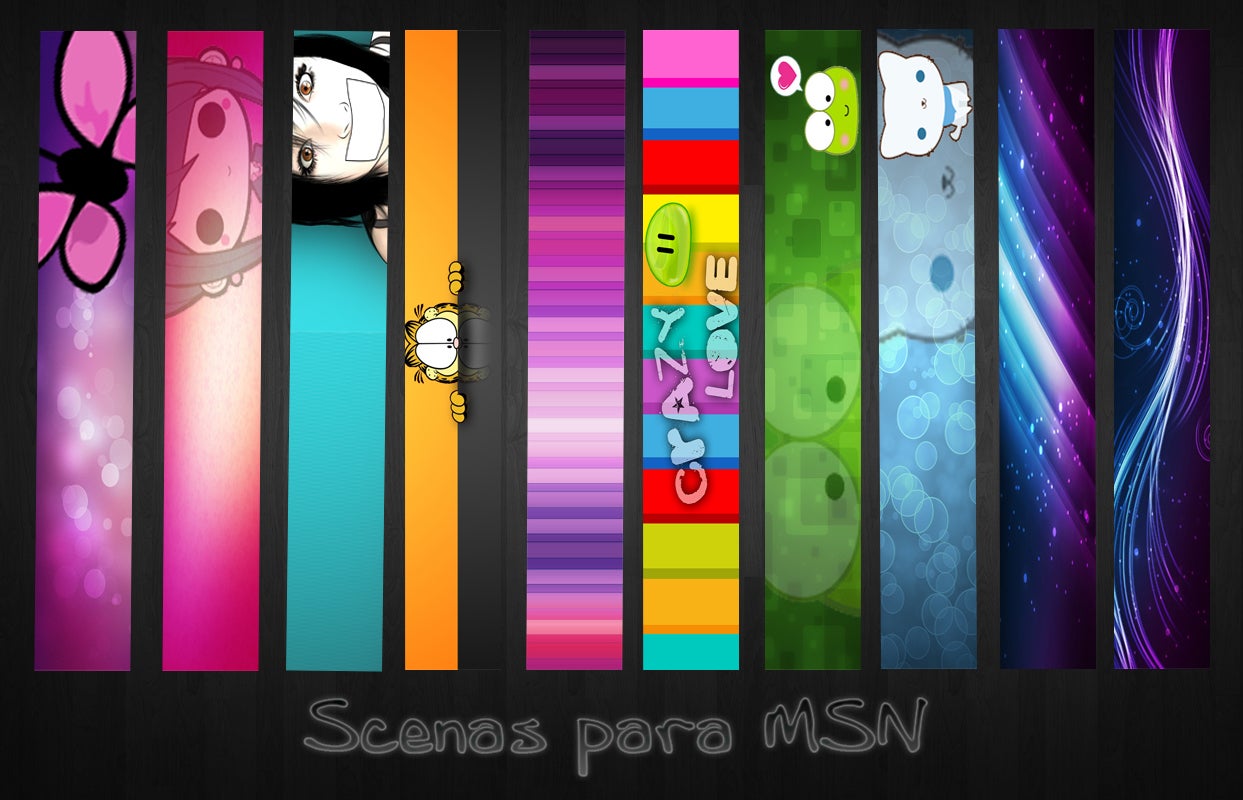The image features ten vertical banners of various designs on a black background. From left to right, the first banner showcases a pink and purple gradient with a black-bodied butterfly with pink wings hovering above white dots. The next banner displays an anime style head of a girl with circle black eyes and blushed cheeks, set against a pink background that lightens towards the center. Following that, another banner features a more realistically drawn anime girl with black hair, brown eyes, white tape over her mouth, and black eyeliner on a blue gradient background.

Moving on, the fourth banner has an orange and black color scheme with Garfield peeking over the black section. The fifth banner is striped with various shades of pink and purple. The sixth banner has multicolored stripes with the text "Crazy Love" and a green blob. The seventh banner presents a smiling frog with blushed cheeks, a heart above its head, set against a green background. Next is a blue banner with a white cat that has blue eyes and a blue collar. The penultimate banner shows a space-themed gradient of purple and blue with some white areas. Finally, the rightmost banner features a fluorescent purple and blue squiggly line running from top to bottom. The text "Sinaspara MSN" is written at the bottom of the image.